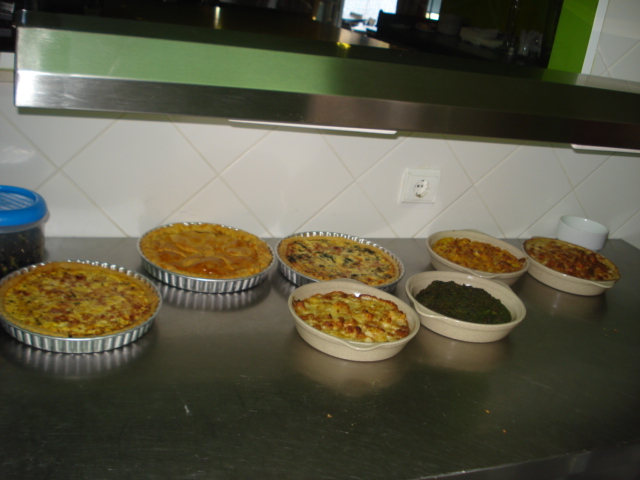This detailed photograph captures a bustling kitchen setting, prominently featuring a stainless steel countertop commonly found in restaurants or bakeries. Spread across the countertop are seven assorted dishes, predominantly characterized as quiches. These dishes are uniquely presented in a variety of pans, ranging from round iron containers and tan ceramic pans to aluminum and clay beige casseroles. Each dish displays a spectrum of colors: some with orangish-yellow hues, others with deep green tones hinting at spinach fillings, one vivid with orangish-red contents, and another with what might be black beans or perhaps a meat dish. On the left edge of the counter, there is a blue-lidded Tupperware container, while on the far right, a single white bowl is visible. The backdrop features a tile backsplash interrupted by an electrical outlet, above which sits a smaller counter bridging the kitchen and server’s area. An overhead metal bar is noticeable, and beyond it, through a window, faint daylight suggests an exterior view or another section of the restaurant.